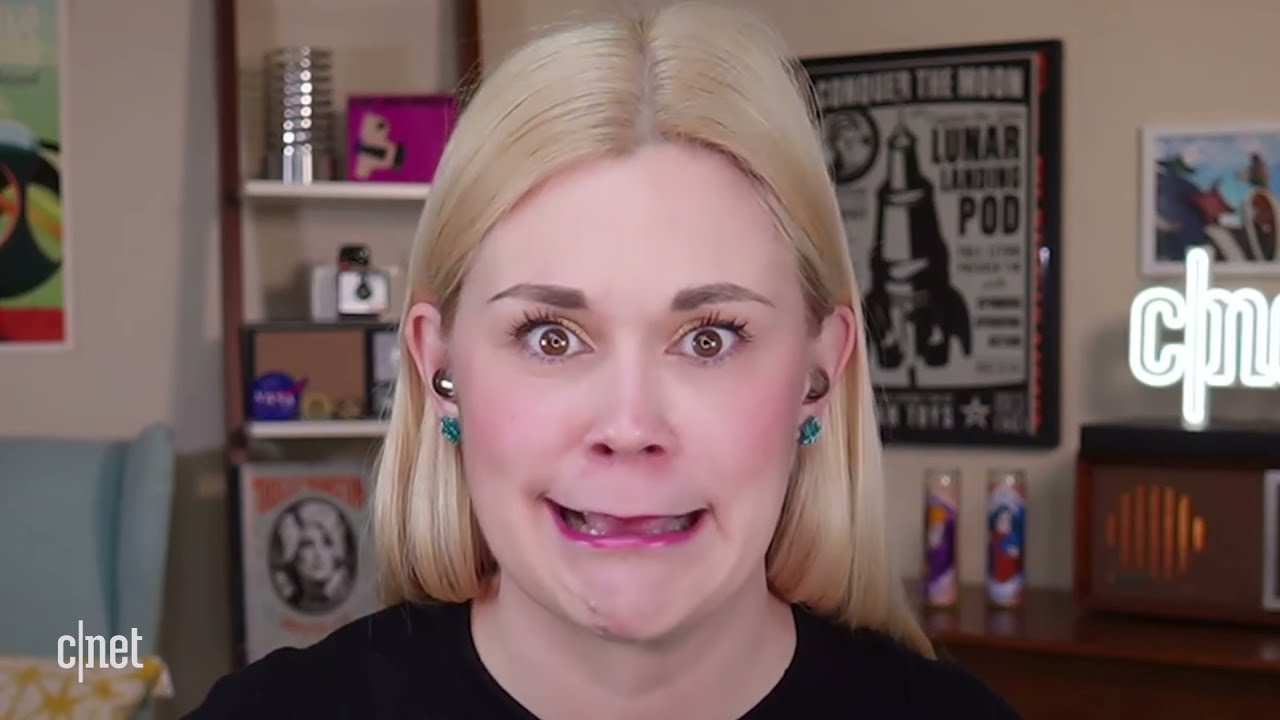This photograph captures a white woman with short blonde hair, wearing green earrings and a black t-shirt, indoors. Her face, framed by short, styled blonde hair, is shown from her shoulders up. She has brown eyes, wide open in a look of surprise or embarrassment, with her mouth slightly agape, forming a crinkly expression. The background reveals a cream-colored wall adorned with pictures, posters, and some shelves holding various objects, including items suggestive of personal interests such as religious candles, a photograph, and even the NASA logo. The lower left corner of the image has a CNET logo in white, hinting that this may be related to an advertisement for a TV show or podcast. The overall scene suggests a snapshot of her living room, providing a glimpse into her personal space.